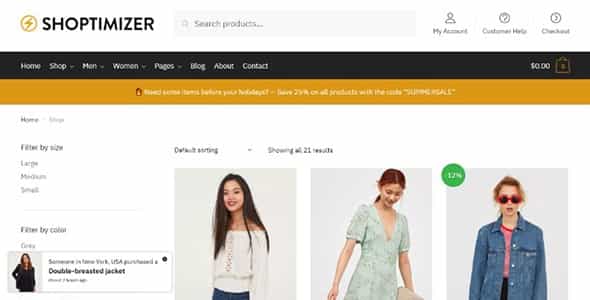**Descriptive Caption:**

This is a screenshot of the Shoptimizer web page. The webpage features a clean, white background. Prominently displayed in the top left corner is the Shoptimizer logo. At the center of the page is a search bar for finding products easily. Aligned to the right are three essential icons: 'My Account,' 'Customer Help,' and 'Checkout.'

Just below this navigation bar, there is a sleek black banner. On the left side of this banner, you'll find clickable categories that include 'Categories,' 'Home,' 'Shop,' 'Him,' 'Women's,' 'Pages,' 'Blog,' 'About,' and 'Contact.' The right side of the banner showcases a shopping bag icon and an amount icon.

Directly beneath this black banner is a horizontal gold-bordered section highlighting a 'Coupon Special Code.' On the right-hand side within this section, there's a small box that includes links to 'Home' and 'Shop.' Below this box, users can filter products by size, with different sizes listed vertically. Similarly, users can filter products by color. There is a pop-up box that provides a thumbnail image and offers inspiration on a specific product.

Moving further down, on the right side of the page, there are three thumbnails displaying models wearing various clothing items, giving customers a visual representation of available fashion pieces.